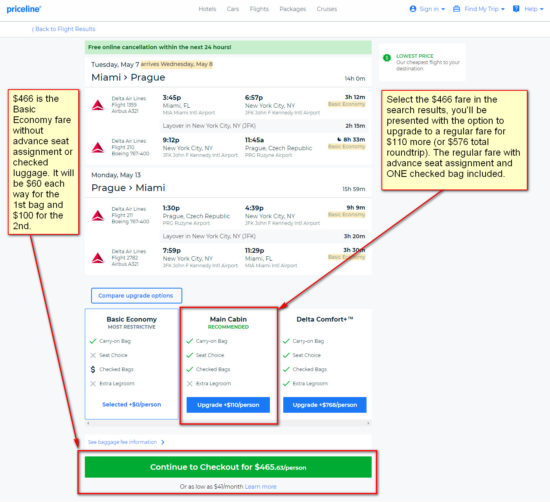This image, captured from the Priceline website, depicts a detailed itinerary for a flight from Miami to Prague. At the top of the screen, there's a section decorated with triangular patterns. Scattered around the page are various annotations, including arrows pointing to different elements of the site.

Prominently displayed is the flight information indicating a departure from Miami, Florida at 3:46 p.m., followed by a layover in New York City from 6:57 p.m. with a two-hour duration until the next leg of the journey. 

On the left-hand side of the image, there's a noticeable yellow box with a red border that outlines the basic economy fare of $466. This fare does not include an advanced seat assignment or checked luggage. Additionally, it states that the first checked bag will cost $60 each way, and the second bag will be $100 each way. 

The page is further highlighted with several other red rectangles and arrows emphasizing certain sections, potentially meant to draw attention to important details or additional information.